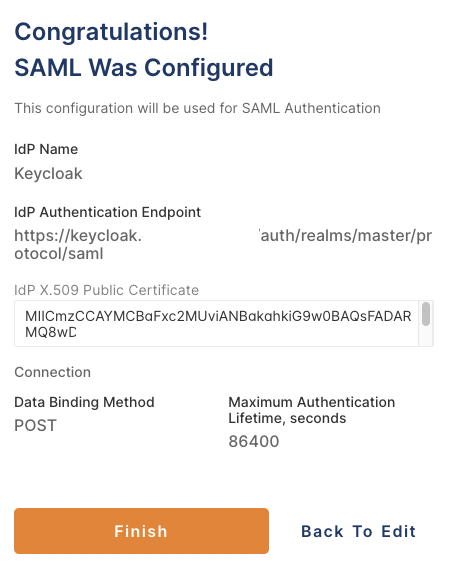The image displays a notification screen within an application interface, primarily set against a crisp white background. The header prominently reads, "Congratulations, SAML was configured," in dark blue or black text. Directly beneath, a subtext elaborates, "This configuration will be used for SAML authentication."

Below the main header, a smaller header labeled "IDP Name" lists "Keycloak" as the Identity Provider (IDP). Further down, another header titled "IDP Authentication Endpoint" is followed by a long URL prefixed with "HTTPS," detailing the specific endpoint for authentication.

An adjacent grayed-out block labeled "IDP X.509 Public Certificate" contains a scrollable text area filled with an extensive string of characters, resembling an encrypted certificate key; a mix of letters and numbers are discernible within.

Continuing downward, a heading titled "Connection" is followed by another heading, "Data Binding Method." To its right, there is a field named "Maximum Authentication Lifetime (seconds)," with the values specified as "Post" for the data binding method and "864,000" seconds for the authentication lifetime.

At the base of the screen, a vibrant orange button with white text stands out, labeled "Finish." Nearby, the text "Back to Edit" in light blue, without an outline but seemingly clickable, completes the interface elements of the image.